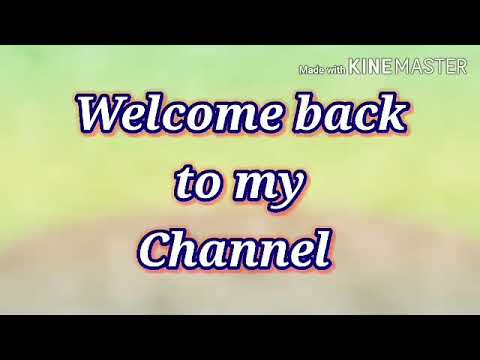The image features a welcoming message with the text "Welcome back to my channel" prominently centered. The text is in white, outlined with a blue border, and accompanied by a pink shadow effect. The background showcases a green hue mixed with gray tones, creating a slightly blurry effect. Towards the top right corner, the text "Made with Kinemaster" is displayed in white, with "kind" notably bold. The image has black borders at the top and bottom, suggesting it is a screenshot, likely from an intro video on a YouTube channel.